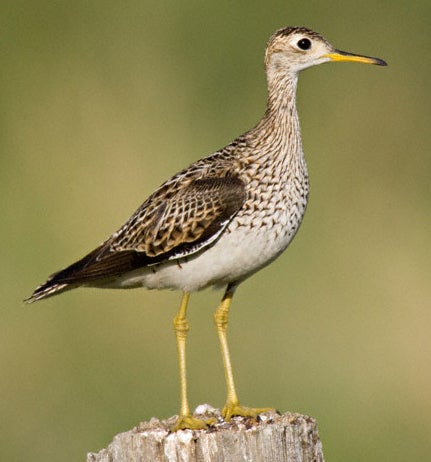The photograph captures a long-legged bird perched on a beige wooden stump against a blurred green background. The bird, centrally positioned and facing to the right, has distinctive yellow and black beak and black eyes. Its long legs are yellow, transitioning into skinny lower limbs with small, possibly webbed feet. The bird's body contrasts its slender legs, being relatively larger, with plumage of mixed colors: brown wings interspersed with white feathers and a white breast extending down its neck. The long neck, though not crane-like, is proportionally elongated for its body size. The wooden stump it stands on is brown, creating a natural perch for the bird within the lush, yet fuzzy greenery in the backdrop.